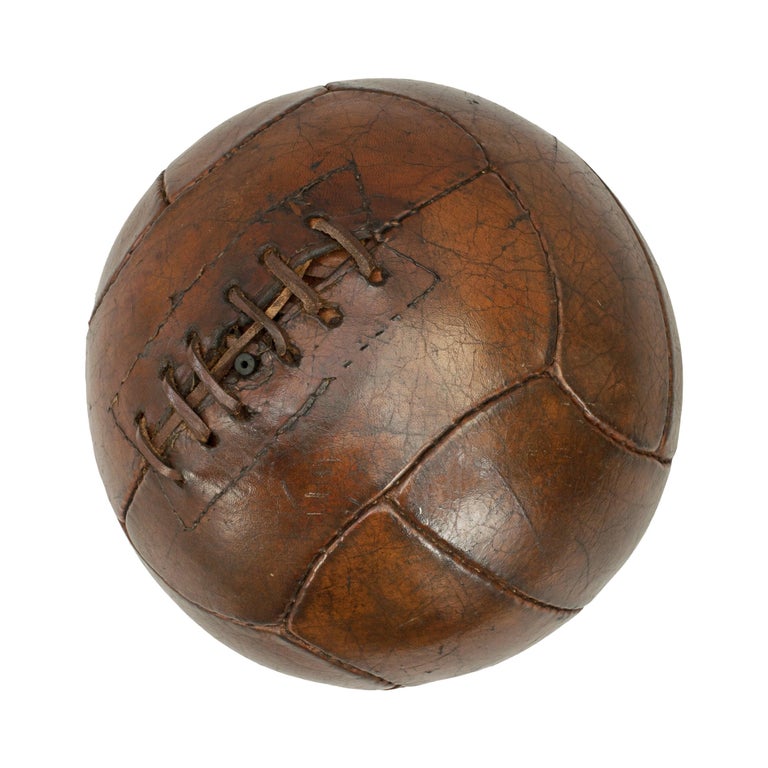A photograph on a white background features an old-fashioned soccer ball made of polished, brown leather. The spherical ball, resembling soccer balls used before the 1960s, is meticulously stitched together from multiple pieces of tanned leather. It showcases a series of prominent leather lacings that resemble those found on a traditional American football but encircle the ball in a round formation. The stitching converges to form a distinct pattern, with six sets of eyelets threaded by rawhide strips that securely hold a replaceable bladder inside. At the center of this lacing, slightly off to one side, is a small black plastic piece with a hole for an air pump needle, indicating where the ball can be inflated. The ball's leather surface is shiny and well-maintained, showing no signs of branding or logos, which adds to its vintage and possibly homemade appearance.